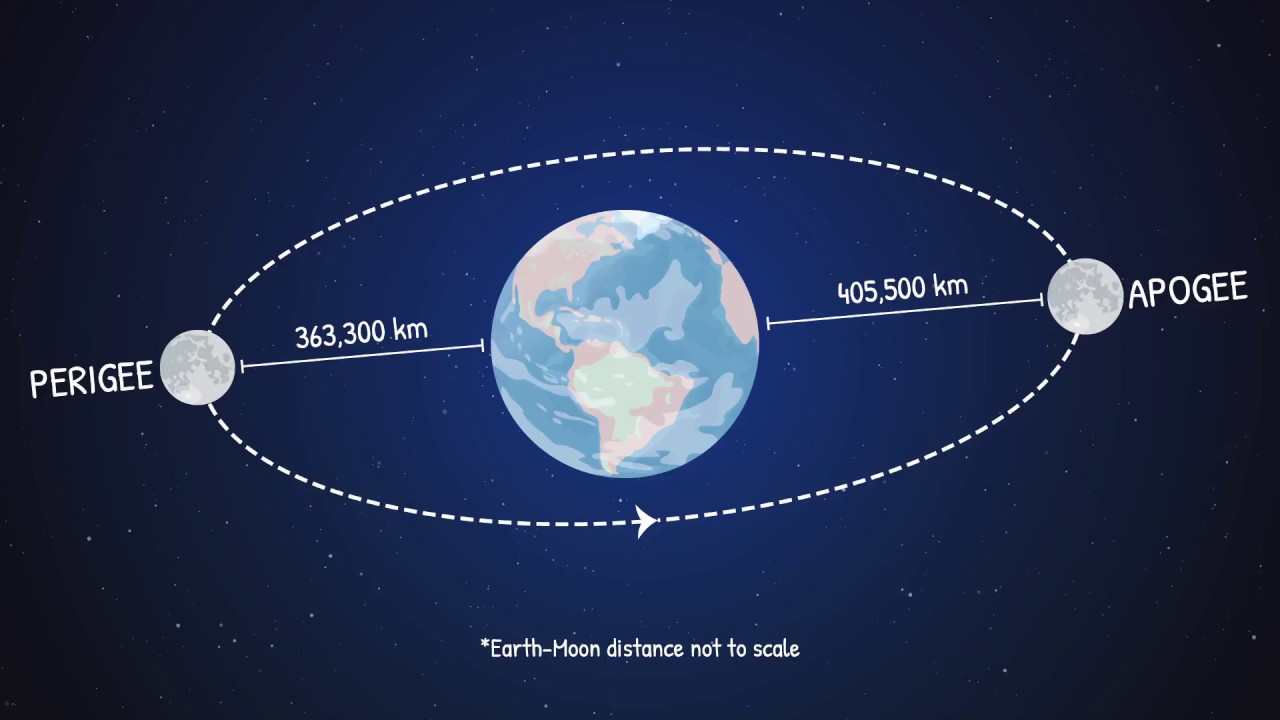The illustration is a detailed, color diagram set against a dark blue, star-speckled background, representing outer space. It features a rectangular, landscape orientation with a depiction of Earth at its center, showcasing North and South America with the oceans rendered in blue and the continents in light pinks and greens, with a small tip of Africa visible to the right. Surrounding the Earth is an elliptical orbit path, slightly tilted toward the bottom left. At the left center of this ellipse is an illustration of the moon labeled “Perigee,” with a white text indication of its distance from Earth as 363,300 kilometers. On the opposite side, diagonally across the ellipse, is another moon illustration labeled “Apogee,” marked with the distance 405,500 kilometers. At the bottom of the image, there is a small note in white text reading “Earth-Moon distance not to scale.”